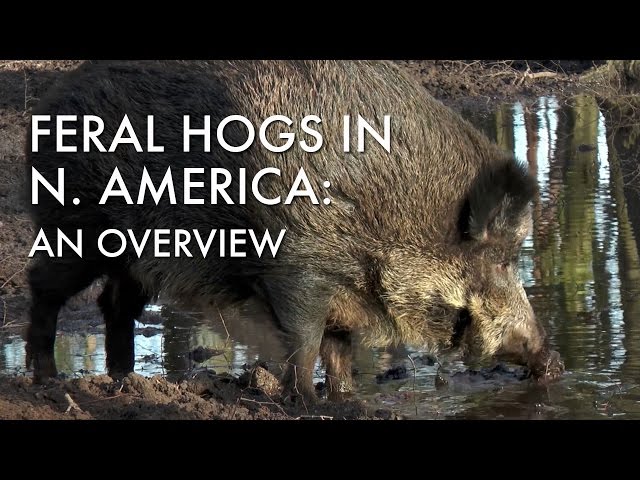The landscape-oriented color image appears to be the title slide of a PowerPoint presentation. Prominent white text at the center of the slide reads, "Feral Hogs in North America: An Overview." Dominating the slide is a close-up profile of a feral hog facing right. The hog is standing in a shallow body of water mixed with clumpy brown dirt or mud. This medium-sized hog sports a coat of varying shades of brown, with a rough texture visible in its fur. Darker fur outlines its round ear, while its snout and neck are a lighter brown, almost tan hue. The animal immerses its snout and nose in the water, seemingly foraging or drinking.